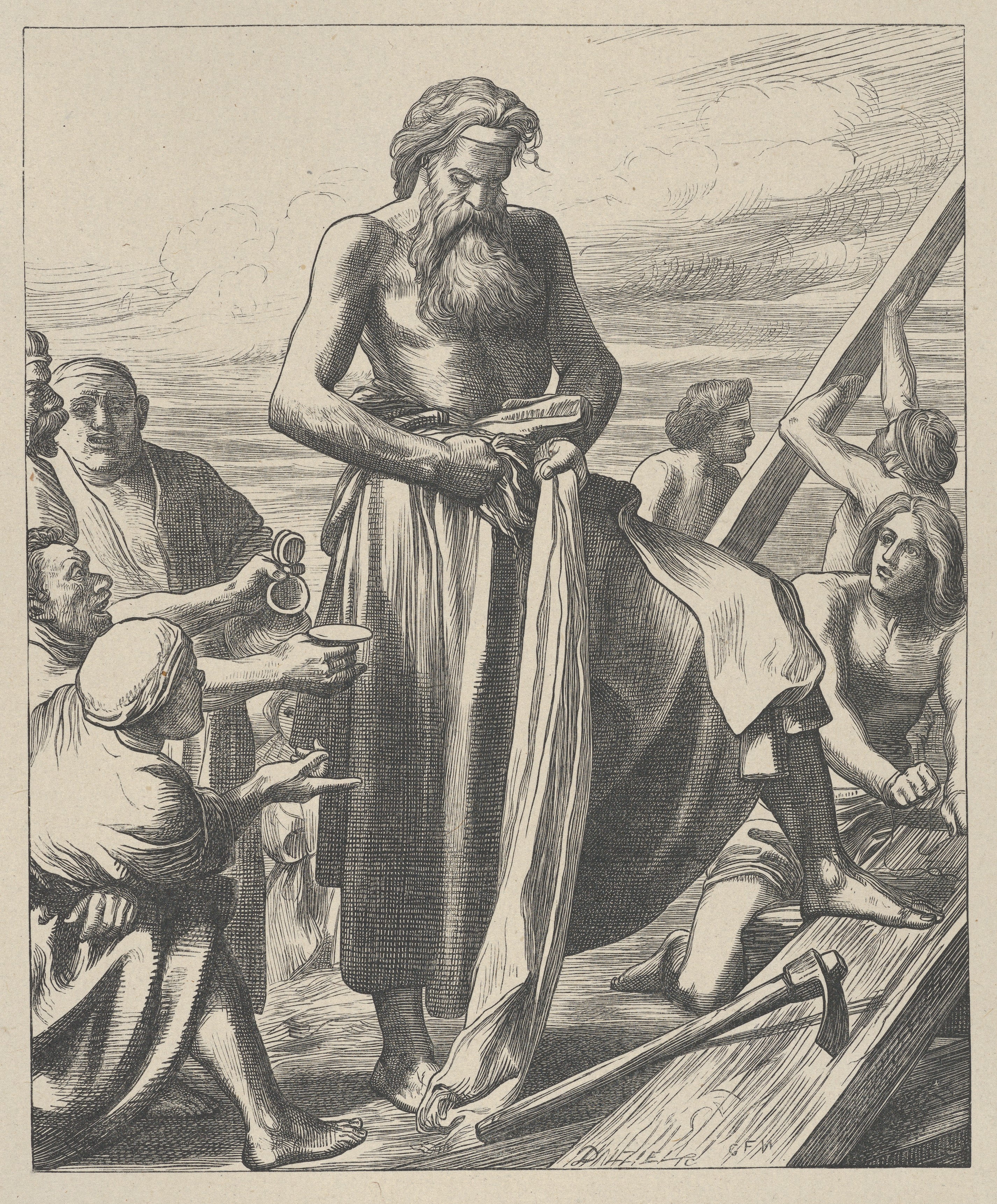This black and white pencil drawing depicts an evocative scene, seemingly set on a boat or near water, as suggested by the faint background elements. The focus is on a central, prominent figure—a man with long, wavy hair and a very long beard and mustache, which reaches the middle of his chest. He is gazing downward, adjusting a wrap or robe tied around his waist, leaving his upper body unclothed. His left foot rests on a large wooden log positioned at the bottom of the image, next to which lies an axe, highlighting a sense of labor or toil. To the man's left are several individuals either sitting or standing, gesturing towards him as if inquiring or pleading. On the right, workers are engaged with wooden logs, with two men holding a plank and another looking up at the central figure. The scene is marked by the serious, somber expressions of all present, evoking a sense of hardship or solemnity. The image is framed by a thin gray line, adding a subtle contrast to the dark cream background, creating an old-world, almost historical atmosphere.